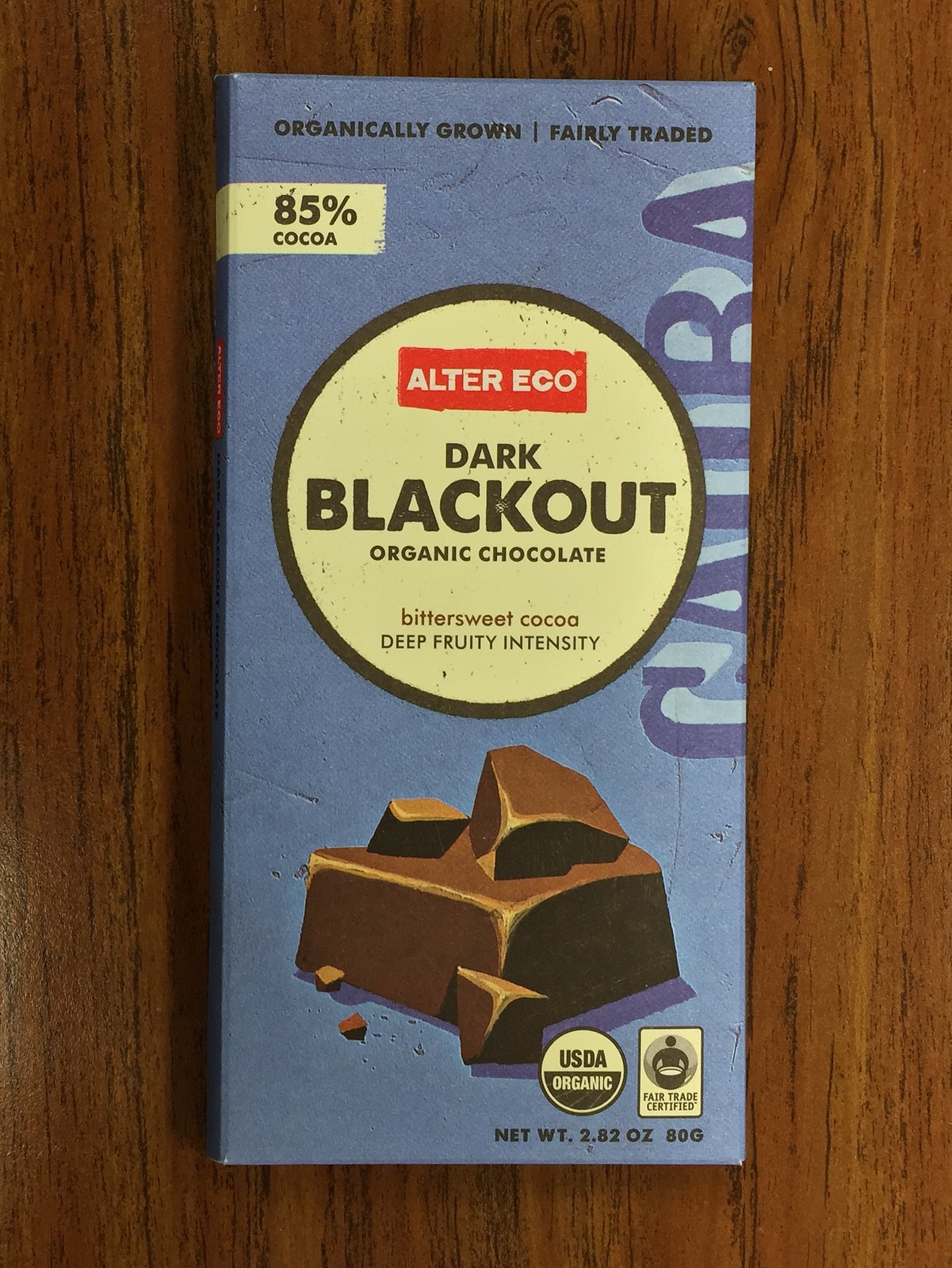The image depicts a chocolate bar resting on a wooden desk or table. The packaging is primarily sky blue and features a well-worn, old-style design, reminiscent of the 1970s or 1980s. At the very top of the package, in small black text, it reads "organically grown, fairly traded," with a small beige banner indicating "85% cocoa." The central focus of the packaging is a large beige-yellow circular section that prominently displays the brand name "Alter Eco, Dark Blackout Organic Chocolate." This section highlights descriptive phrases such as "bittersweet cocoa" and "deep fruity intensity." Below this circle, there's a red banner with white text repeating "Alter Eco," and an illustration of chocolate chunks just beneath it. To the right of the illustration are certifications including the "USDA Organic" stamp and a "Fair Trade Certified" label. The net weight is specified at the bottom as 2.82 ounces (80 grams). The chocolate's presentation emphasizes its organic and fair-trade qualities, aligning with its trustworthy and premium branding.